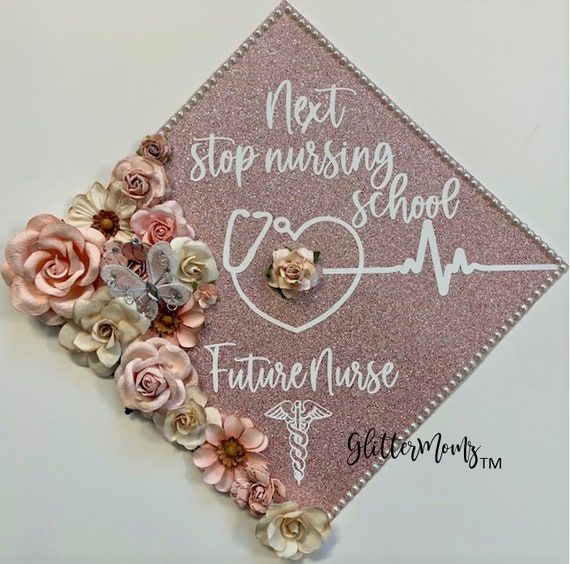This image captures a beautifully decorated graduation cap, meticulously crafted with significant detail, likely as a gift for an aspiring nurse who has just graduated high school and is headed to nursing school. The cap, tilted to resemble a diamond shape, is adorned with a sparkly lilac background inscribed in elegant cursive with the phrase, "Next Stop Nursing School." Below, in similar cursive, it reads "Future Nurse," accompanied by the classic medical symbol of a snake wrapped around a rod with wings.

A standout feature of the cap is a heart cleverly formed from the cord of a stethoscope, symbolizing both love and the medical field. Pulsing lines emerge from the heart, giving the design dynamic energy. At the center of the heart is a delicate rose, adding a touch of softness.

The cap is intricately embellished along its edges with a mix of pearl-like beads and a variety of 3D flowers, including muted colors of pink, blue, ivory, and tans. This arrangement features roses and sunflowers, contributing to a rich, floral aesthetic. Additionally, a light blue silk butterfly graces the left-hand side of the cap, enhancing its whimsical look.

The cap bears the trademark "Glitter Mom's," suggesting a personalized or handcrafted touch. The backdrop is a clean, white surface, presumably to highlight the cap's detailed and thoughtful decoration.